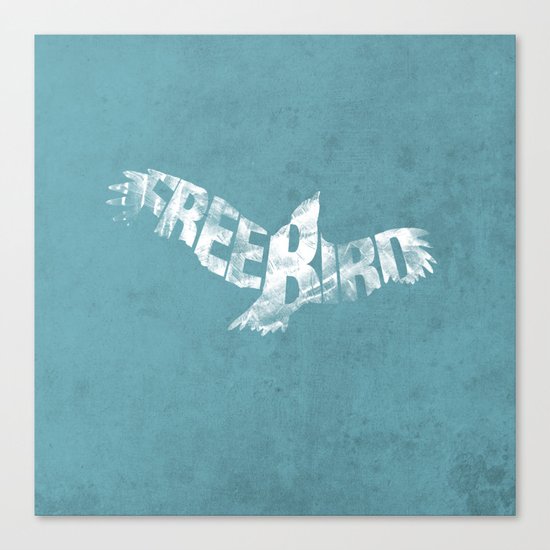This image, resembling an album cover, features a vertically rectangular design set against a white background. The cover itself is characterized by a matted teal blue (or prismarine) color, with slight variations in shading, lending depth with soft specks of gray and black. Dominating this teal blue canvas is an artistic rendering of a bird, which appears to be created using splotchy, incomplete white paint, revealing traces of the teal background through it. This bird's wings are outstretched and it gazes upward, perhaps toward an unseen sun. Intriguingly, the bird's shape is constructed entirely of the letters forming the words "FREE BIRD," with each part of the bird's anatomy corresponding to a different section of the text: the left wing reads "F-R-E-E," the body forms the letter "B," and the right wing completes the image with "I-R-D." The overall aesthetic suggests a graffiti or print style, capturing a sense of artistic freedom and homage to the famous song "Free Bird" by Lynyrd Skynyrd.